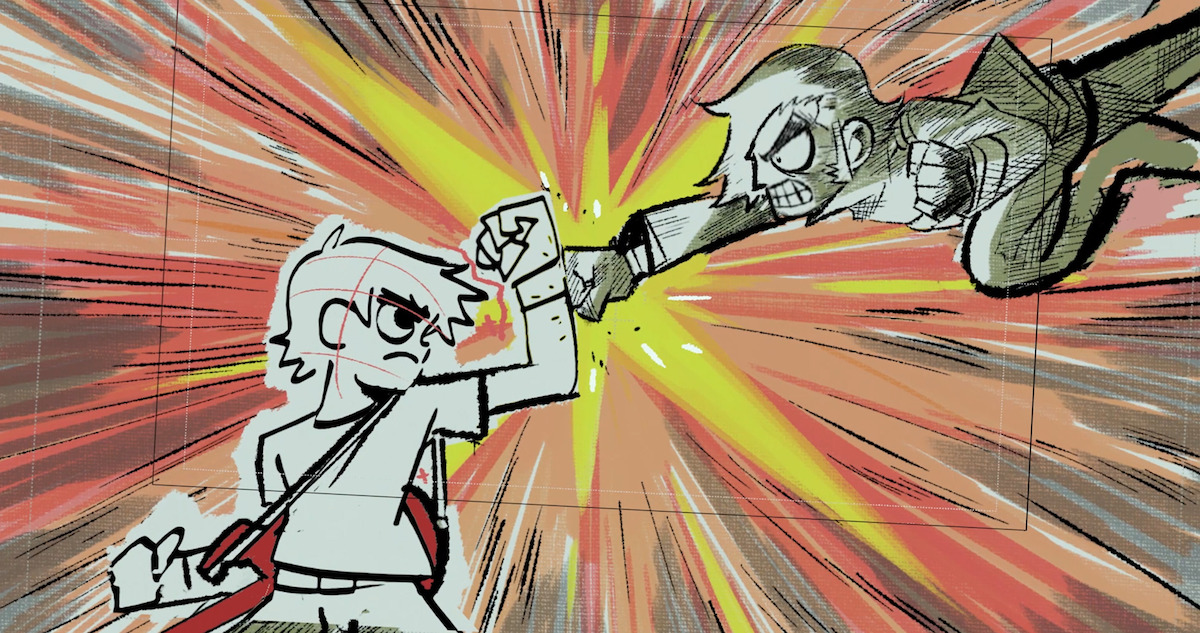The image is a colorful illustration, reminiscent of the Scott Pilgrim series, horizontally oriented and detailed like a comic strip panel. It features two distinct characters with black pencil outlines. To the left center, there's a character resembling Scott Pilgrim, who is all white with a red guitar strapped to his back, blocking a punch with his left hand. The attacking character emerges from the top right-hand portion, drawn in shades of white and dark greenish-tan, and appears to be very angry, his teeth gritted as his fist makes contact with Scott's wrist. From the point of impact, a dynamic explosion of light radiates outward. This action-packed burst, resembling a BAM POW star, features a kaleidoscope of colors—pastel orange, red, brown, yellow, and a multitude of reds and grays, creating an intense, spiraling energy. Surrounding the two characters is a light frame of white and black, highlighting the confrontation. The background includes speed lines and flashes, adding to the vivid sense of motion and action.